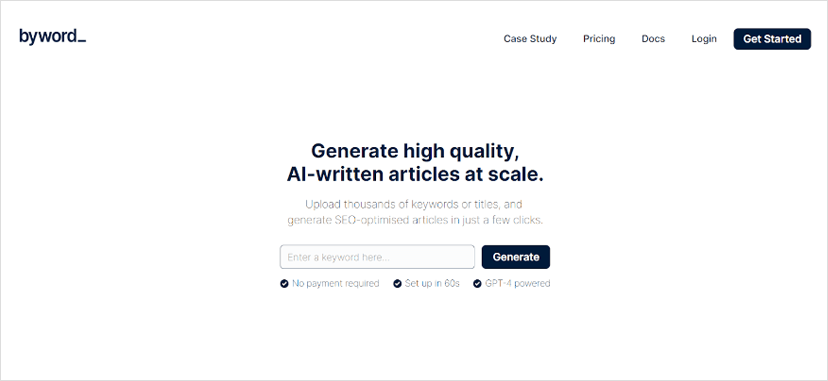Here is the cleaned-up and detailed description for the screenshot of the advertisement:

The screenshot features an advertisement on a white background. In the upper left corner, the text "buy word..." is displayed in black font. On the right side, there are navigation options in black font that read: "Case Study," "Pricing," "Docs," and "Login." Below these options is a prominent black rectangle with the white text "Get Started."

At the center of the screen, in bold black font, the phrase "Generate High Quality AI Written Articles at Scale" is prominently displayed. Beneath this, a subtitle in light gray font reads: "Upload thousands of keywords or titles and generate SEO optimized articles in just a few clicks."

Underneath the subtitle, there is a gray input rectangle with the text "Enter a keyword here." To the left of this input field is a black button with the white text "Generate."

In the lower left corner, three features are listed, each accompanied by a black checkmark: 
- "No payment required"
- "Set up in 60 seconds"
- "GPT-4 powered"